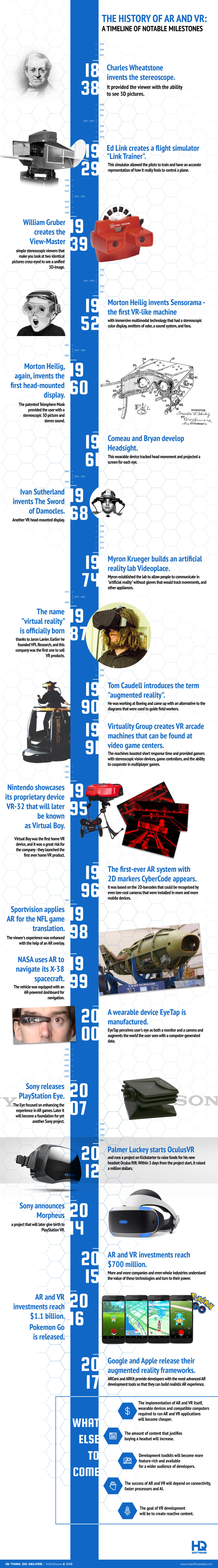The image portrays a vertically oriented, highly condensed timeline, approximately half an inch wide by seven inches tall, illustrating the evolution of ocular and visual devices from 1838 through to 2017 and beyond. Dominating the timeline is a prominent blue stripe that runs from top to bottom, flanked by a series of small, alternating images and accompanying text, though the text is too minuscule to read without magnification. The timeline begins with an image of a stereoscope viewer, accentuating significant milestones such as the View-Master from 1939. As the timeline progresses, it features a variety of visual devices, leading up to modern VR headsets around 2007 to 2012. Among the diverse imagery, one can identify objects like a ship reminiscent of the Titanic, a blimp, a fighter jet, a red object, and what appears to be a figure resembling Einstein near the top. Despite the detailed visual elements, comprehending the finer points of the text requires a closer look or zooming in.